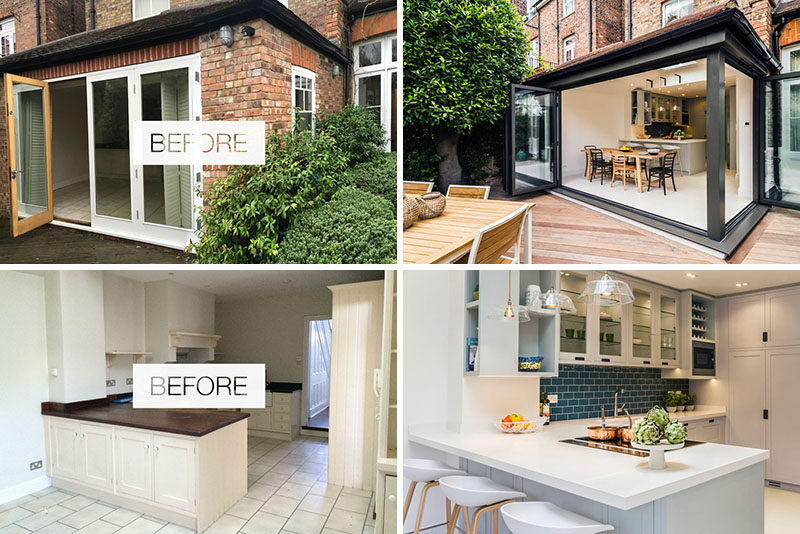This collage-style image is divided into four quadrants, with a clear distinction between 'Before' (left side) and 'After' (right side) transformations of a house. The top two quadrants feature exterior shots of a house's back patio. The 'Before' image on the top left shows an enclosed brick patio with a white-bordered French door leading outside and a black-roofed structure surrounded by shrubs. The 'After' image on the top right displays a modernized open patio with sliding glass doors that fully open to reveal a chic kitchen and dining area.

The bottom two quadrants showcase the kitchen's transformation. The 'Before' image on the bottom left depicts a dated, mostly white kitchen with plain white cabinets, dark brown countertops, and white tile flooring. In contrast, the 'After' image on the bottom right highlights an updated and more inviting space. The cabinets are still white but now feature glass fronts, the countertops are a sleek white, and a striking blue tile backsplash has been added. The kitchen is further illuminated by trendy pendant lights and enhanced with a revamped bar area featuring three stools. Each before image is marked with a white rectangle and the word 'BEFORE' in transparent text, emphasizing the dramatic changes made.